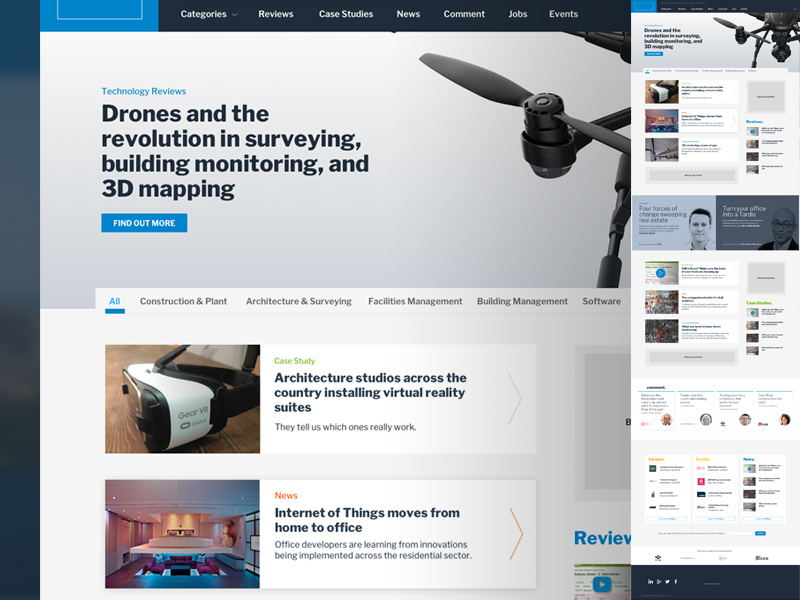The image features a visually intricate layout dominated by various shades of blue and black, and is divided into several distinct sections with specific content.

On the far left side, there is a dark blue vertical strip running down the length of the image. The topmost section of the image includes a light blue square. Below this, a black segment features different categories such as “categories, reviews, case studies, news, comment, jobs, and events” inscribed within it. Another light blue section follows, interspersed with more black areas that contain minuscule writing.

Central to the image is a gray background that showcases the title “Technology Reviews” in blue font and highlights the theme “Drones in the revolution in surveying, building, monitoring, and 3D mapping,” accompanied by a blue “Find Out More” button below a flying drone image.

Beneath this, there’s a light blue box with underlined text reading “All”, followed by category labels: "construction and plant," "architecture and surveying," "facilities management," "building management and software." Adjacent to this, there are two square images. The first square, labeled “Case Study” in green, mentions “Architecture studios across the country installing virtual reality suites. They tell us which ones really work” in blue text on a white background, accompanied by a right arrow. The second square, titled “News” in red, states “Internet of Things moves from home to office. Business developers are learning from innovations being implemented across the residential sector,” with a red right arrow.

Following these squares, another section in gray features the heading “Review” in blue, a card with a green line and a blue square inside it.

On the far right, the uppermost box on a light blue background repeats the drone image and a blue button, accompanied by three small images and another gray square with smaller images. Below this, a segment depicts two men in colored boxes—one light blue and the other dark blue—followed by three white-background boxes. There’s a gray box with a single word and four small pictures lining the side, leading to a gray button.

The bottom portion of the image transitions to a white background containing four small pictures of people and their comments, followed by another white box divided into three columns filled with pictures and icons. At the very bottom, a blue button and a final stretch of gray conclude the detailed layout.